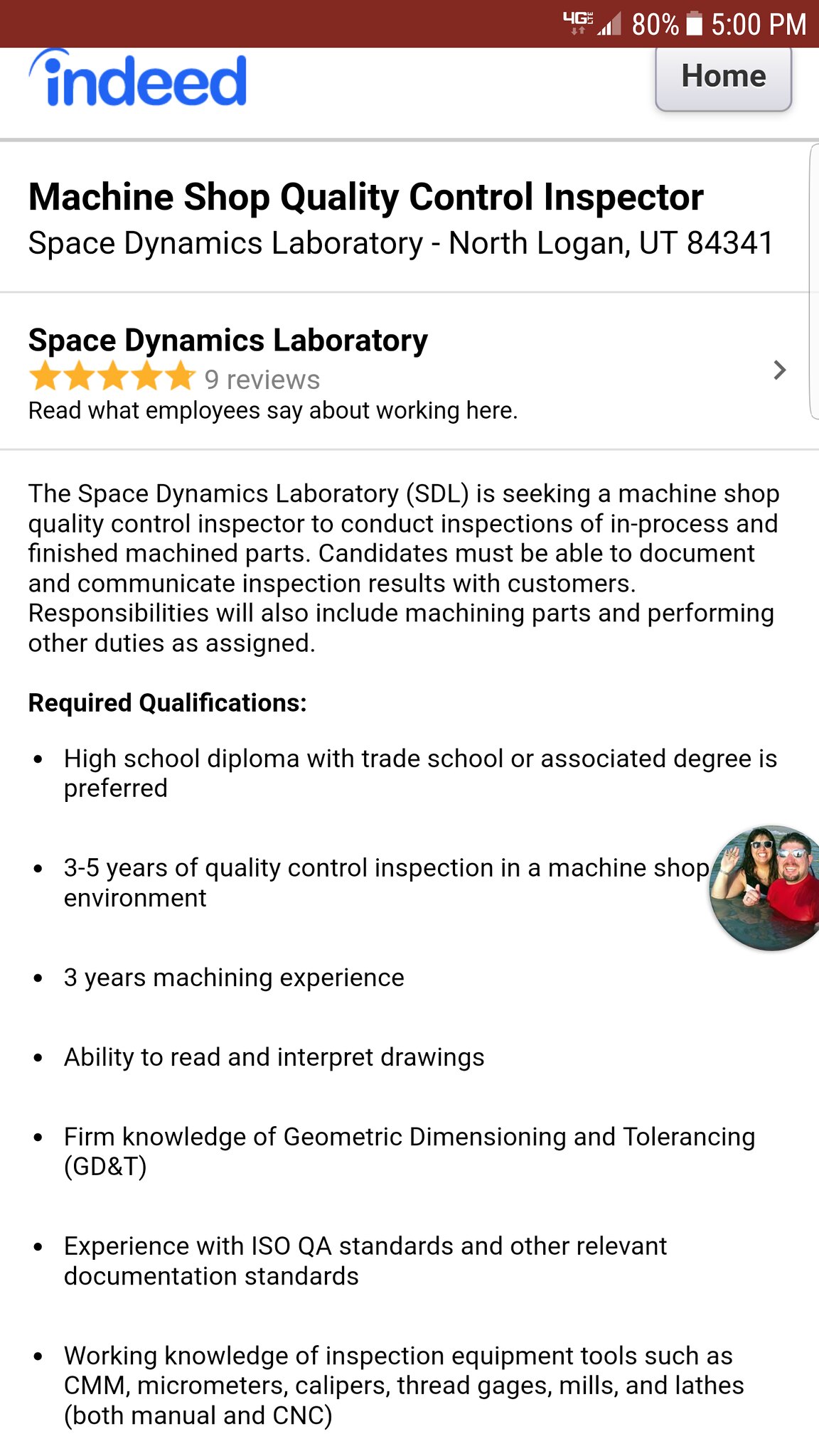The image is a screenshot of a detailed job listing on the Indeed website, viewed on a mobile phone. At the very top is a maroon border displaying the battery life at 80%, the time at 5 p.m., and other phone indicators. Below this, the word "Home" appears on the right, and "Indeed" in blue text appears on the left. The primary job posting is for a "Machine Shop Quality Control Inspector" at the Space Dynamics Laboratory in North Logan, Utah, 84341. The listing includes a four-gold-star rating from nine reviews. 

The job description details that the role involves conducting inspections of in-process and finished machine parts. Candidates must document and communicate inspection results and perform other machining and related duties as assigned. The text is set against a white background with blue, black, and yellow gold elements highlighting key information. 

Additionally, towards the middle right is a full-color photograph of a man and a woman, both wearing dark sunglasses. The detailed qualifications for the job run down the page, emphasizing the extensive descriptive nature of the job posting.